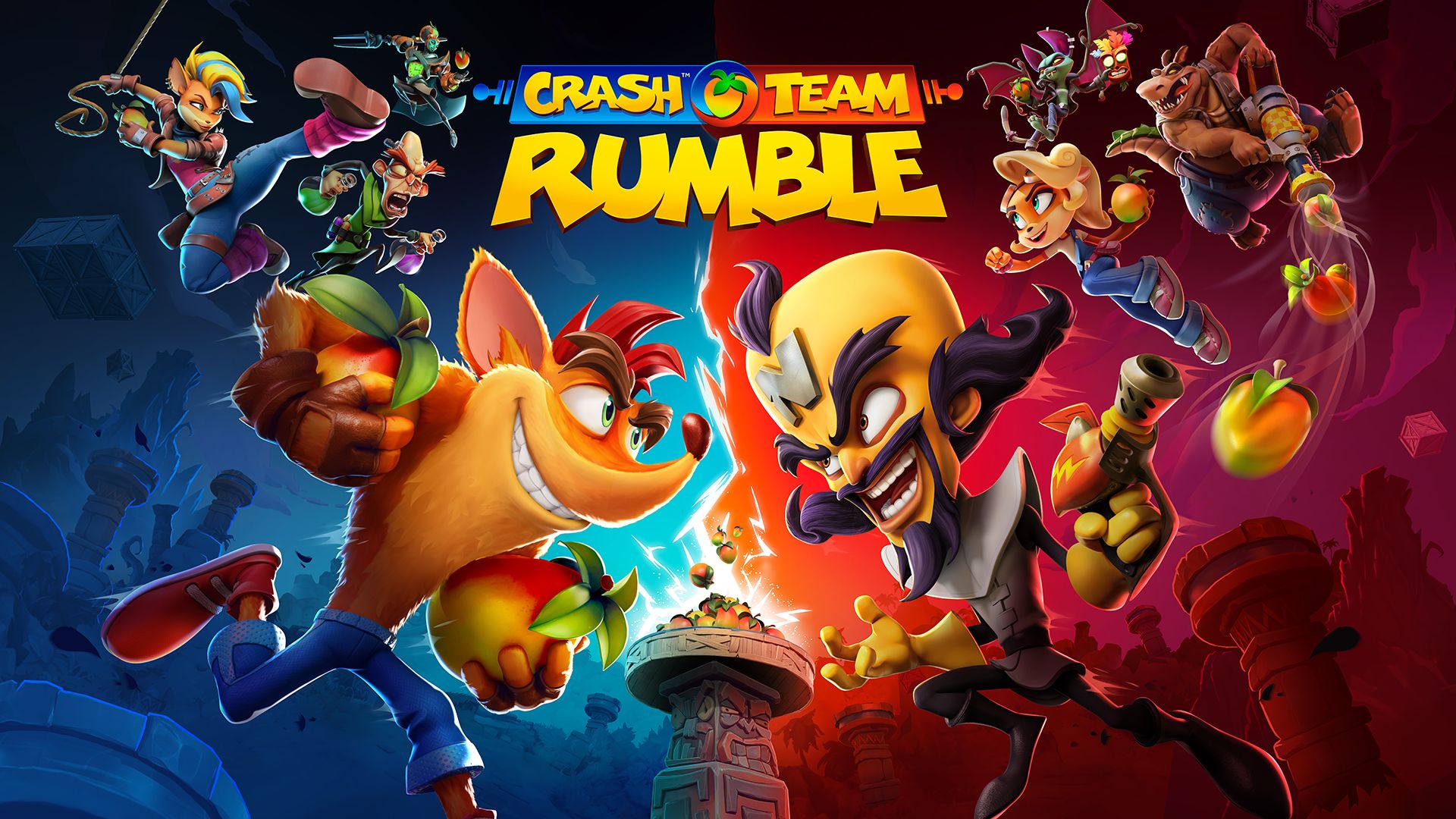The image is a vibrant and action-packed banner graphic for the game "Crash Team Rumble," designed to capture the energetic essence of the game. Dominating the top center is the game title in a dynamic layout, with "Crash" in bold yellow text on a blue background, "Team" in matching yellow on a red background, and "Rumble" underneath in funky large white letters.

The central scene is divided by a striking electric bolt, symbolizing the intense clash between the characters. On the left half, set against a blue background, is the iconic Crash Bandicoot, a cartoonish orange-furred creature sprinting forward with two mango-like Wumpa Fruits in his hands. Behind him, three smaller allies appear engaged in the action.

On the right half, featuring a reddish-purple background, stands the menacing Neo Cortex, identifiable by his oversized head, a goatee, sinister curled eyebrows, and a signature 'N' on his forehead. He wields a ray gun and is flanked by three smaller henchmen. Between the two factions, Wumpa Fruits appear to be electrified, possibly on an Aztec-like pedestal, adding to the dramatic showdown vibe.

The major colors in the image are vivid and diverse, including shades of orange, red, blue, green, black, white, yellow, and gold, all contributing to the high-energy atmosphere of the scene. The overall composition underscores the head-to-head competition with an elaborately detailed and colorful depiction of the game's characters and their epic rivalry.